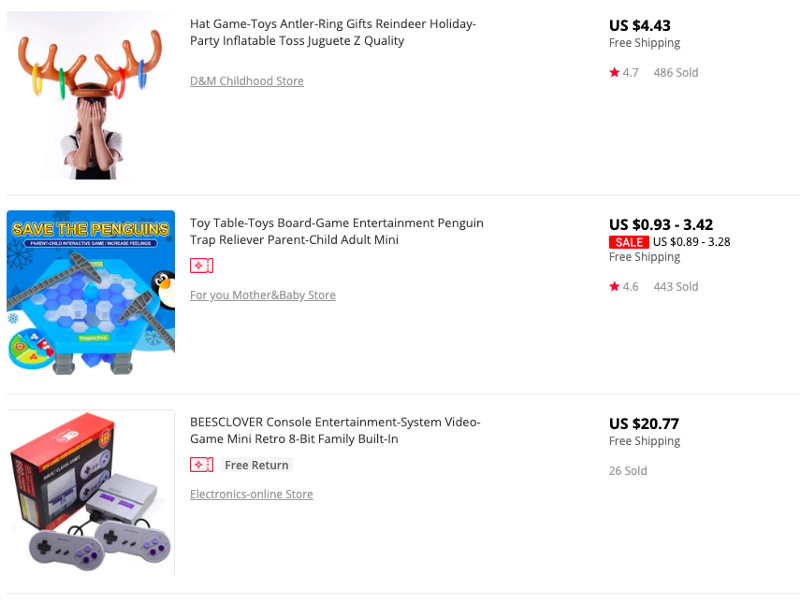This image showcases an e-commerce website with a white background, featuring items for sale. On the left side of the image, there are pictures of the items. Centrally located are the names of the items, and on the far right side, there are details including pricing, star ratings, the number of units sold, and information about free shipping.

The first item displayed is a "Head Game Toys Antler Ring Reindeer Holiday Party Inflatable Toss," priced at $4.43 with free shipping. The next item is a "Toy Table Board Game Penguin Trap Reliever," with a price range from $0.93 to $3.42 and also free shipping. The last item listed is a "Console Entertainment System Video Game Retro 8-Bit," priced at $20.77 with free shipping, and it has 20 units sold.